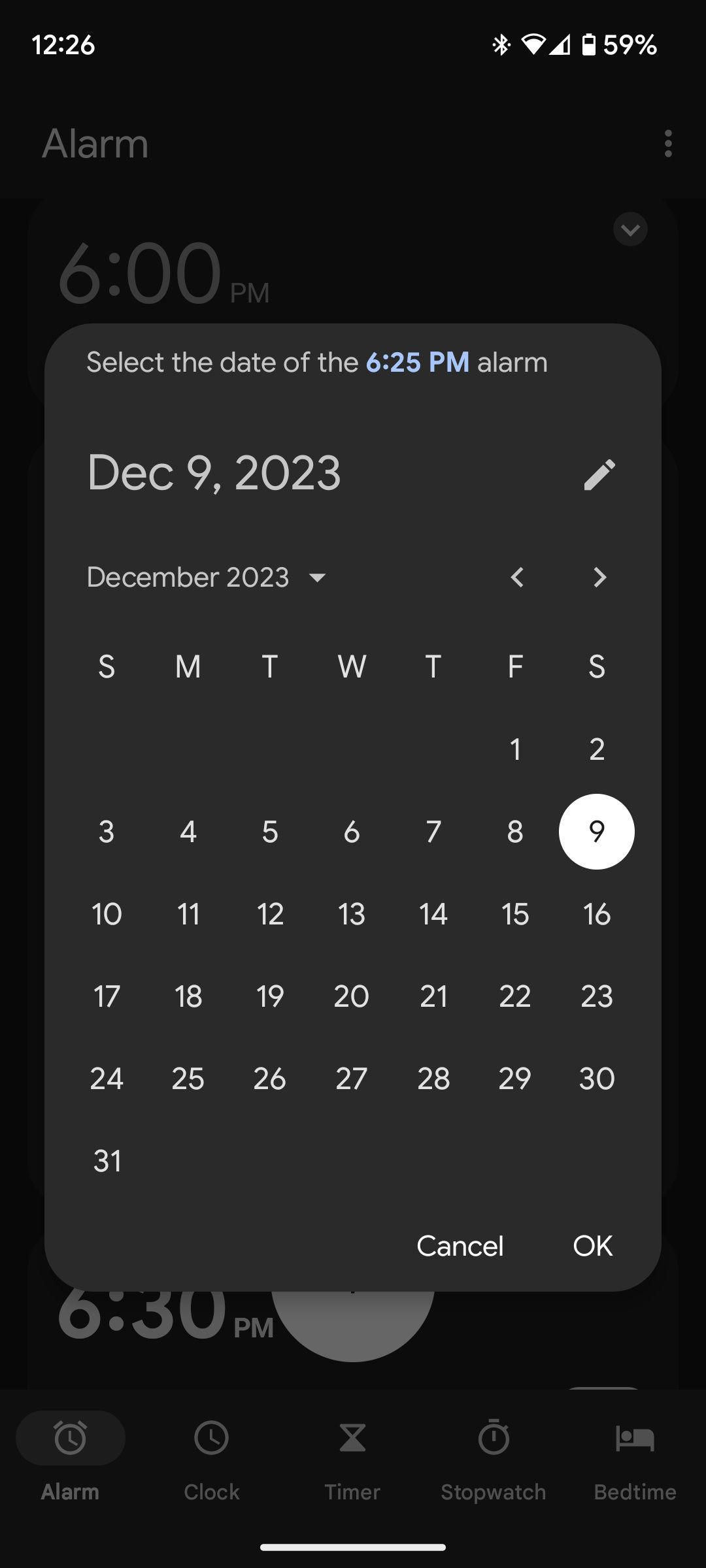A screenshot capturing a smartphone user's calendar interface. The device displays a black background, with the status bar at the top left showing the time as 12:26, and to the right, icons for Wi-Fi, battery status (at 59%), and an alarm indicator with three dots beside it. Below this, '6:00 PM' is listed as one of the set alarms. Dominating the screen's center is a pop-up calendar selecting the date for a 6:25 PM alarm. The date December 9, 2023, is highlighted in blue, and a pencil icon for editing appears to the right. The calendar layout for December 2023 is visible, with days 1 through 31 clearly marked and the current selection, December 9, highlighted with a white circle. At the bottom of the pop-up, there are 'Cancel' and 'Okay' buttons. The base of the screen features navigation options: Alarm, Clock, Timer, Stopwatch, and Bedtime.